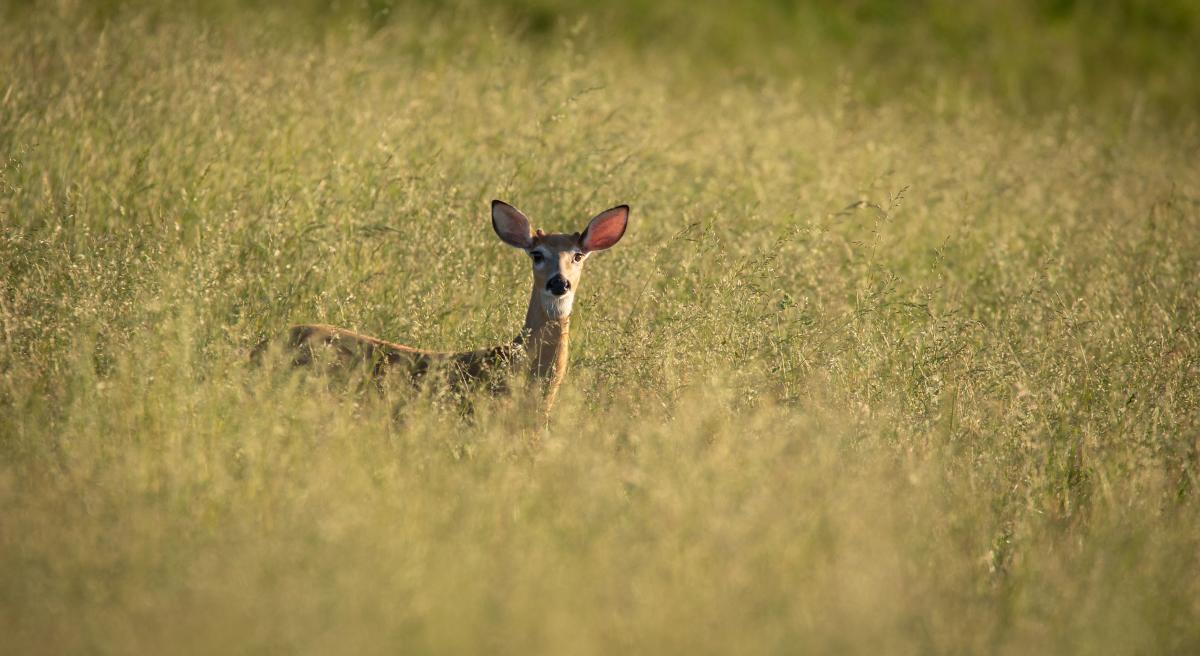In this captivating photograph, a young deer stands amidst a field of tall, yellowish-green grass, which blurs around the edges, drawing focus to the deer at the center. The deer's body is tan, with its light-colored or white face, neck, and distinctive features standing out sharply. Its alert, large ears are directed towards the viewer, with the sunlight filtering through the left ear, creating a striking pinkish-red hue due to the veins. This deer is likely startled, having just looked up from grazing as the photographer made a sound, prompting it to freeze and gaze directly into the camera. The sunlight softly illuminates the right side of its face, accentuating the detailed textures of its fur and the expressive black eyes, complemented by the white markings around its eyes and muzzle. This serene and somewhat monochromatic image captures the quiet vigilance and beauty of the deer in its natural habitat during what appears to be an afternoon.